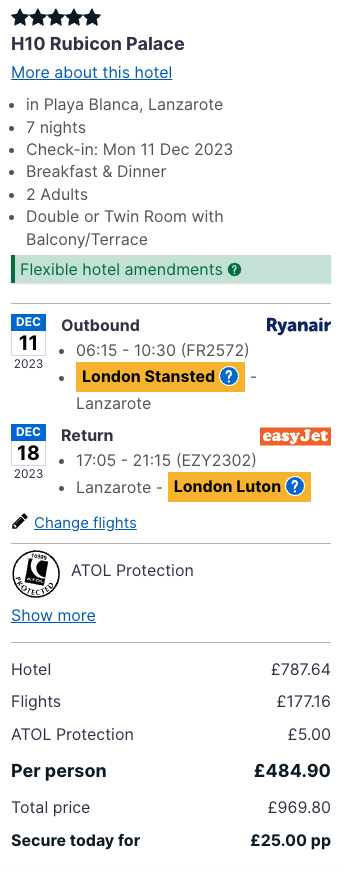On a pristine white background, five black stars are positioned in the top-left corner, signifying a high-quality rating. Next to the stars, the text reads "H10 Rubicon Palace." Below that, in blue and underlined, is the phrase "more about this hotel." 

In gray text, the following details are listed:
- Location: Playa Blanca, Lanzarote
- Duration: Seven nights
- Check-in date: Monday, 11 December 2023
- Meal plan: Breakfast and Dinner
- Occupancy: Two adults
- Room type: Double or Twin Room with Balcony or Terrace

A green banner highlights the phrase "flexible hotel amendments," accompanied by a circle with a question mark. Below this, a fine gray line separates sections of information.

A blue and white calendar icon displays "December 11" with "2023" and flight details:
- Outbound: 06:15 to 10:30
- Flight number: FR2572 (Ryanair)
- Departure airport: London Stansted, denoted by a blue circle with a white question mark
- Destination: Lanzarote

Another blue and white calendar icon shows "December 18, 2023," and return flight details:
- Return: 17:05 to 21:15
- Flight number: EZY2302 (EasyJet)
- Departure: Lanzarote
- Destination: London Luton, highlighted with an orange banner with "EasyJet" in white

An option to "change flights" is presented in blue, underlined text with a pencil icon signaling the ability to edit. Another fine gray line follows this section.

Underneath, "ATOL protection" is noted with a black-outlined circle and the word "protected." A "show more" option is also available in blue, underlined text, followed by another fine gray line.

The pricing breakdown is detailed as:
- Hotel: £787.64
- Flights: £177.16
- ATOL protection: £5 per person, totaling £10
- Final total: £969.80

Additionally, it mentions "secure today for £25.00 pp" (per person).